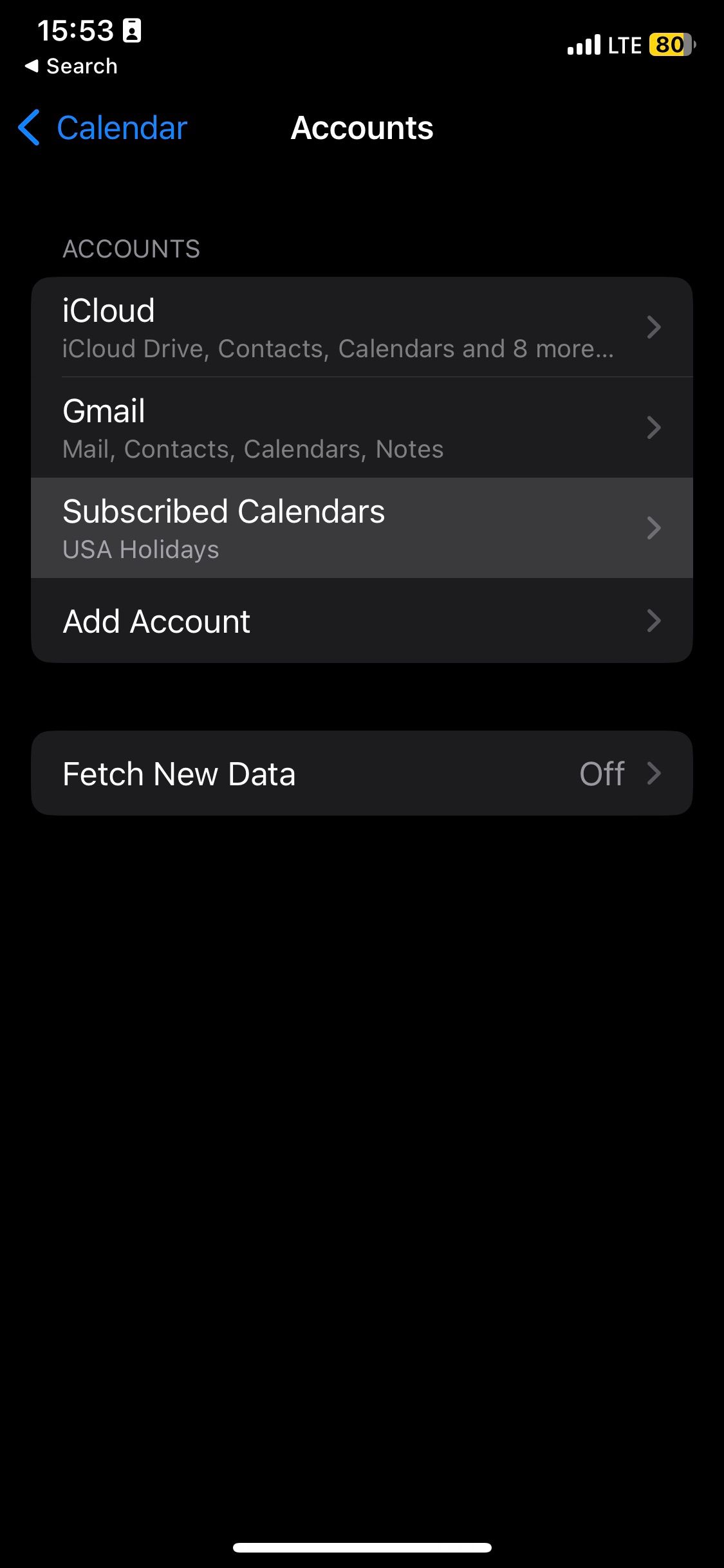This image is a screenshot of the Settings app on an iPhone, specifically within the Accounts section. The screenshot was taken at 15:53 and shows that the user is connected to LTE with a strong signal and has an 80% battery level. At the very top of the screen, there is a small "Search" icon with an arrow pointing to the left, followed by a blue-highlighted "Calendar" label, also with an arrow pointing to the left.

Central to the image is the "Accounts" heading, below which various account options are listed. The first option is "iCloud," which is detailed as including iCloud Drive, Contacts, Calendars, and eight other items, with an arrow indicating further details can be accessed. Next is "Gmail," encompassing Mail, Contacts, Calendars, and Notes, also expandable with an arrow.

Following Gmail, "Subscribed Calendars" are displayed, currently listing only USA Holidays, with an option to add more. The "Add Account" section provides an arrow for adding additional accounts. Finally, the "Fetch New Data" setting is shown as toggled off but includes an arrow for modifications.

The interface includes a grab bar at the bottom, suggesting the screenshot is from a recent iOS version likely in dark mode, as indicated by the black background.